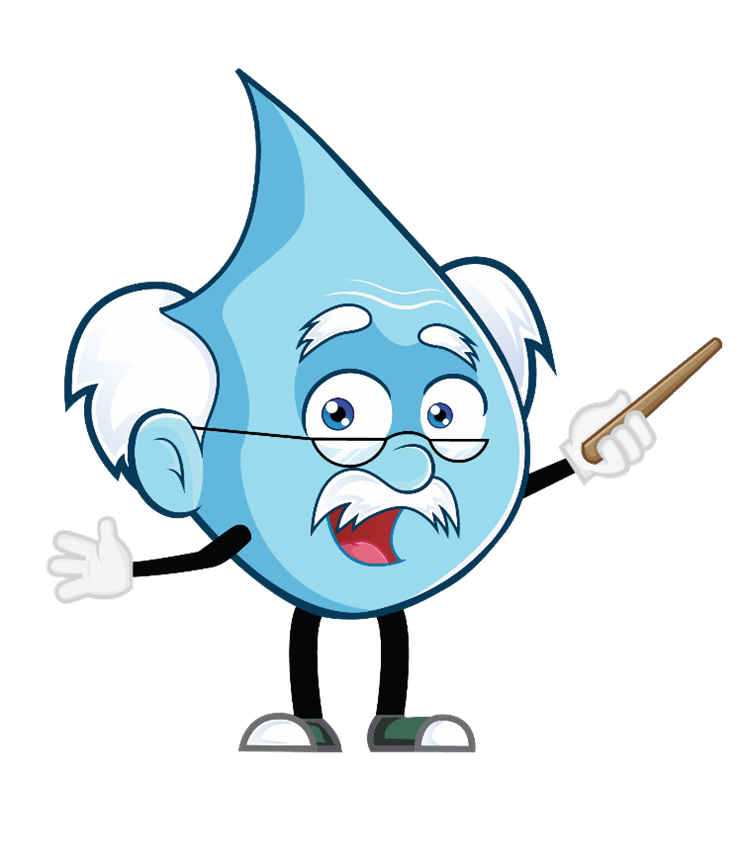The image is a detailed illustration logo featuring a cartoon character with a humanoid teardrop shape that represents a knowledgeable, elderly man, possibly an interpretation of Albert Einstein as a drop of water. The character is predominantly blue and has a teardrop-shaped head that serves as its entire body. Tufts of white hair sprout from the sides, accompanied by bushy white eyebrows, a gray mustache, and half-rimmed reading glasses perched above his blue eyes. The character has cartoonish, skinny black limbs and wears white gloves with three fingers and a thumb, echoing the style of Mickey Mouse. He sports little white and green sneakers on his feet. In one hand, he holds a pointer stick, suggesting he is in the act of teaching, his mouth open with a bright pink tongue visible as if he's speaking. The background is plain white, emphasizing the vibrant and educational nature of this eccentric, professor-like water drop character.